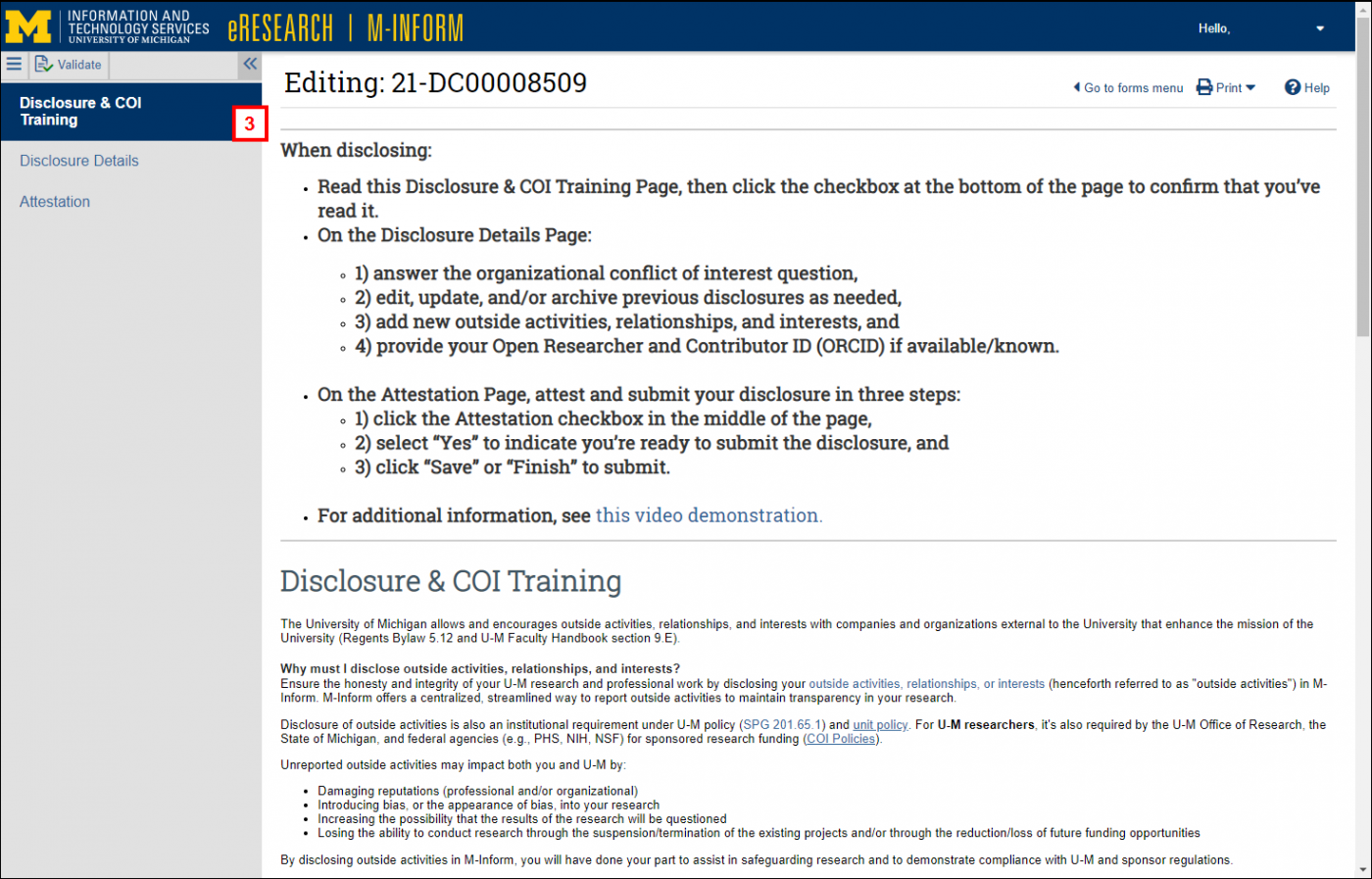At the top of the image, there is a yellow "M" logo, followed by the text "Information and Technology Services University of Michigan" in white font. Next to it, the words "eSearch" and "M inform" appear, all set against a navy blue background. 

Below the "M" logo, three horizontal lines are visible, accompanied by the word "Validate." Additional text reads "Disclosure and COI training," alongside a red box containing the number "3" in white.

The section below includes the labels "Disclosure," "Details," and "Attestation." In the top-right corner, the word "Hello," followed by a comma, and a white down arrow are displayed.

The central part of the page contains a section of text indicating, "Editing 21 DC 0008509." Instructions are provided, stating: "Once closing, please read this Disclosure and COI training page, then click the checkbox at the bottom of the page to confirm that you've read it."

Further directions outline the steps for the "Disclosure, Details" page:
1. Answer the organizational conflict of interest question.
2. Edit, update, and/or archive previous disclosures as needed.
3. Add new outside activities, relationships, and interests.
4. Provide your Open Researcher and Contributor ID (ORCID) if available or known.